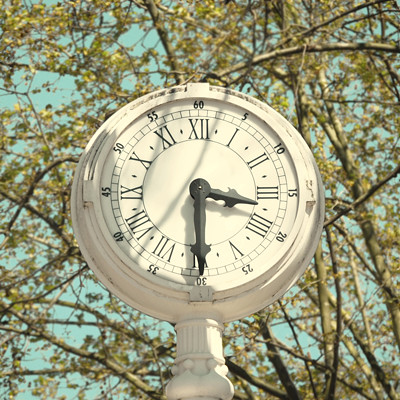A square-shaped image captures an outdoor clock set against a picturesque backdrop. The background features a vibrant blue sky partially veiled by trees with brown stems and green and yellow leaves. The clock, circular and white, prominently stands in the foreground. It displays both standard and Roman numeral black numbers, along with sleek black hands that mark the time against its clean, contrasting face.